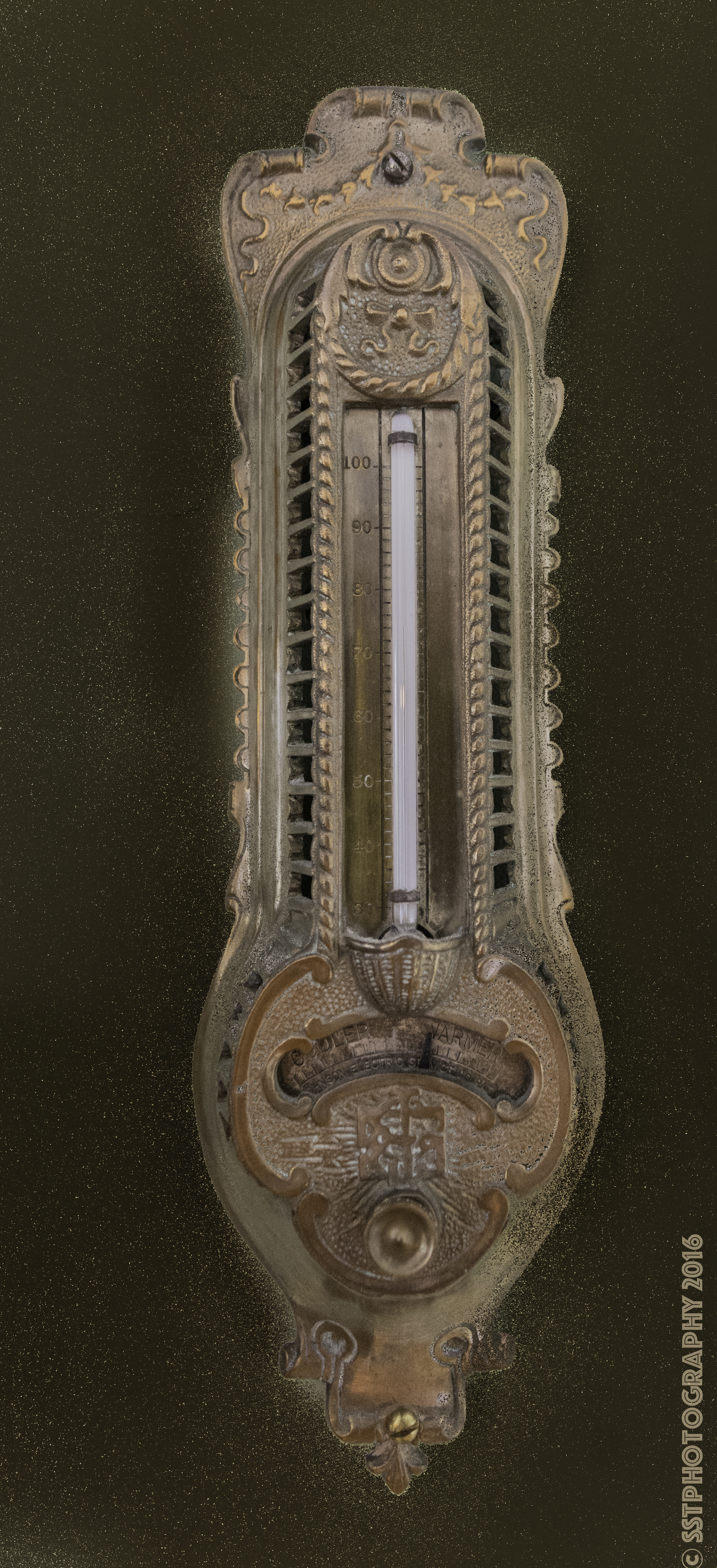This tall, narrow photograph appears to be taken for an eBay-style listing, showcasing a potential antique brass scale. The object is meticulously placed against a dark brown backdrop, likely a table, enhancing its intricate details. The scale, constructed entirely of brass, exudes a vintage charm with its ornate decorative accents.

At the center of the scale is a long, narrow gauge, predominantly white, marked with various weight increments. The clearly visible top marking reads "100," with subsequent tick marks indicating different weight measurements, such as 80 or 90. Although the functional hook part of the scale is not visible, the detailed craftsmanship and brass screws contribute to its aesthetic appeal. The combination of the brass and the contrasting white gauge make it a striking piece that hints at its historical utility and elegance.